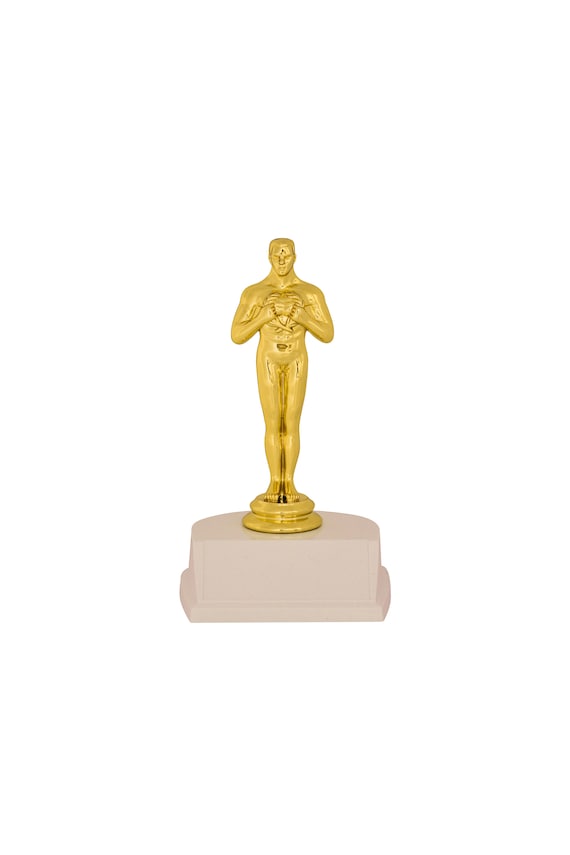The image depicts a gold-colored figurine that closely resembles an Oscar award, adorned with specific features. The statue showcases a man with broad shoulders, short hair, closed eyes, a defined nose, and a mouth. Uniquely, the man has his arms bent with his hands raised in front of his chest, seemingly forming the shape of a heart, evoking an image suggestive of Superman opening his chest. His legs are long, feet are detailed with toes, and he stands on a distinctive half-moon and square-shaped base that is light brown in color. The backdrop of the image is a plain white background, highlighting the intricate details of the figurine. The design of the trophy seems significant and possibly commemorative, reflecting the emotional resonance awards like the Oscars carry, celebrating major accomplishments and special moments with fans and families.